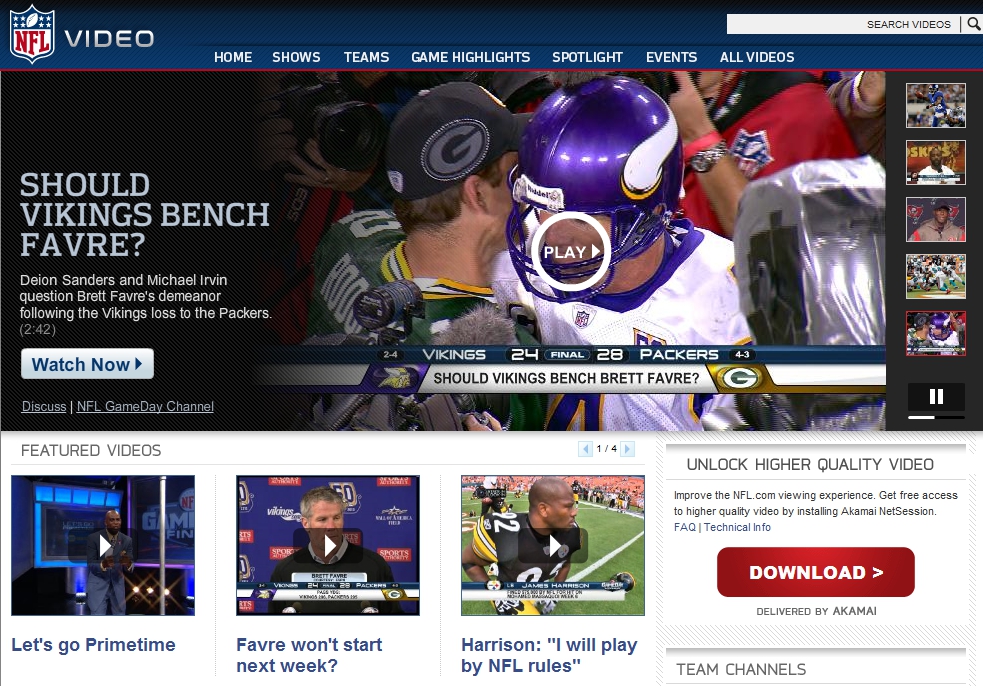This is a detailed screenshot of the official NFL website. In the top left corner, there is the NFL shield logo, featuring a small football above the red letters "NFL." To the right of the logo is a blue bar running across the top of the page, containing a "Video" link. The search bar is positioned on the top right, labeled "Search Videos."

Below this blue bar is a navigation menu featuring options: Home, Shows, Teams, Game Highlights, Spotlight, Events, and All Videos. Dominating the next two-thirds of the screen is a large central image showing two football players in an embrace. One player is a white man with short brown hair, wearing a black hat with the letter "G" on it and a green jersey with yellow and white accents; his name, which starts with "R-O-D" or "R-O-O," is partially visible. He is giving a hug to another player who is also white, with a purple helmet adorned with white horns, indicating he is likely a member of the Minnesota Vikings. This player is wearing a white jersey with a purple letter on the front.

In the foreground, there is a camera wrapped in plastic to protect it from rain, and a microphone with a fuzzy cover positioned close to the two players. On the left side of the image, a title reads, "Should Vikings bench Favre?" followed by a subtitle, "Deion Sanders and Michael Irvin question Brett Favre's demeanor following the Vikings loss to the Packers." Information about the video's length (2 minutes 42 seconds) is shown, along with a "Watch Now" button, and tabs labeled "Discuss" and "NFL Game Day Channel."

Below the hugging players and script, the score "Vikings 24 Final 28 Packers" is prominently displayed. On the right side of the screen, there are five clickable video thumbnails, including two featuring men being interviewed at a table. Beneath the main image are three larger video thumbnails. The first shows a man in a blue suit standing, with the caption “Let's Go Primetime.” The second thumbnail features Brett Favre in an interview setting with an NFL-branded background panel, captioned “Favre Won't Start Next Week?” The third thumbnail depicts a bald black man wearing a Green Bay Packers jersey number 22, with the quote “I Will Play By NFL Rules – Harrison.”

At the bottom of the screenshot, there is an option to download and unlock higher quality video.